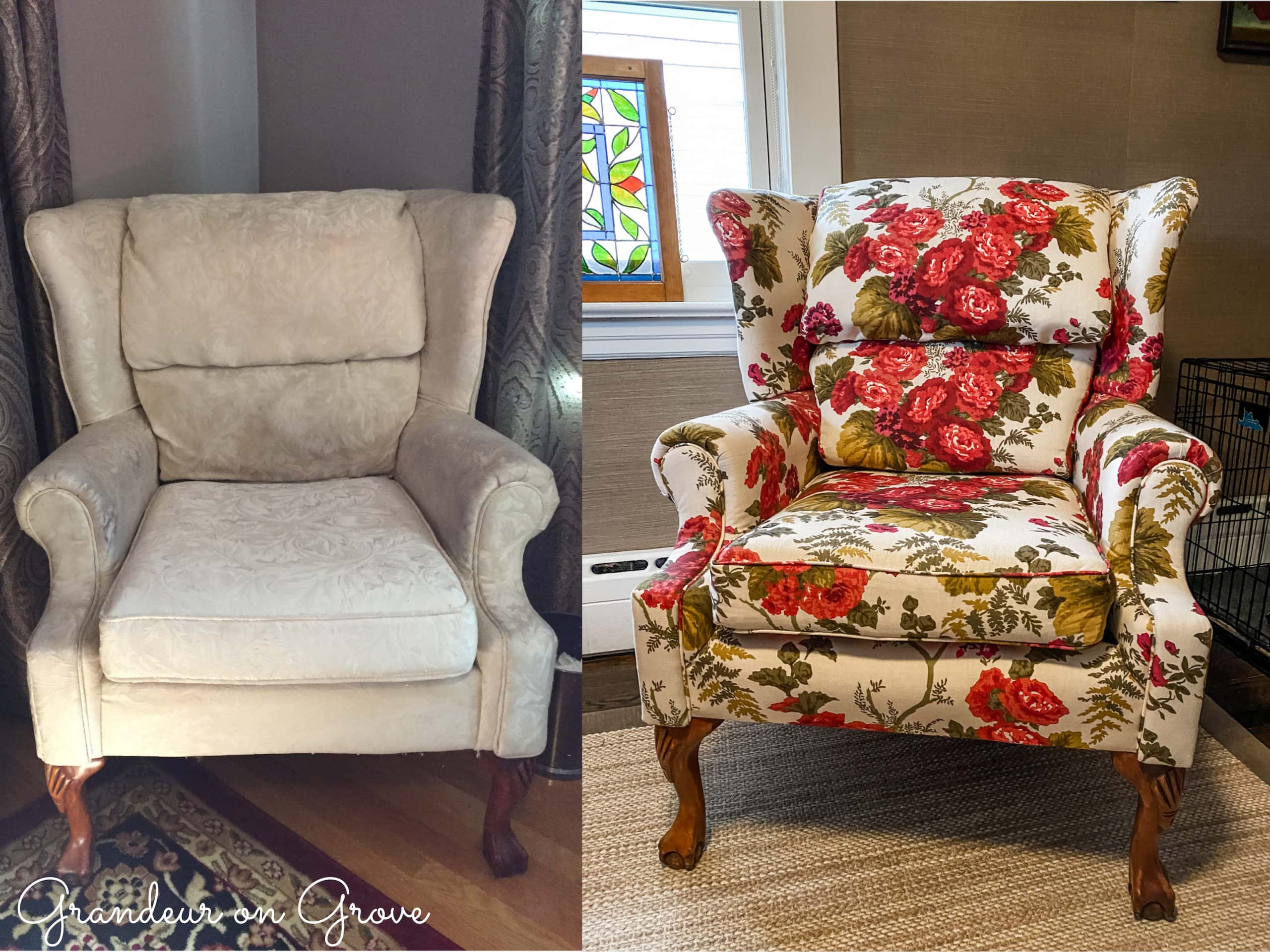The square image comprises two vertically rectangular, full-color photographs presented side-by-side to show a before-and-after transformation. In the bottom left-hand corner, the text "Grandeur on Grove" is written in white cursive. 

The left photograph features an Old-style chair with wooden, pedestal-style legs and a backrest with winged flares that envelope the sitter's head. The chair is upholstered in a worn-out, cream-colored fabric with subtle imprints and lacks decorative flair. It sits in a dimly lit room. 

In contrast, the right photograph displays the same chair, now refurbished and reupholstered with a vibrant floral fabric. The new upholstery showcases a bright white base decorated with vivid green leaves, vines, and bold red roses, giving the chair a refreshed and elegant appearance. The setting also changes, placing the chair in a more brightly lit room with a large window in the upper left corner, highlighting the transformation's dramatic effect.